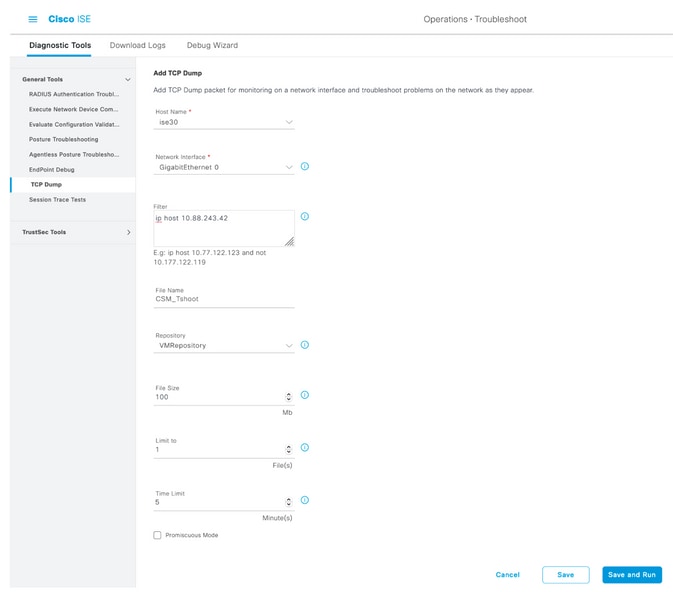Certainly! Here’s a cleaned-up and highly detailed caption for the image:

---

**Detailed Description of an Online Settings Page**

This screenshot captures an online settings page, organized in a roughly square format with distinctive sections and headers. The page layout features a left panel, occupying approximately 20% of the image, with a dark light gray background, and a right main body with a white background, devoid of borders on the bottom and right sides.

**Header Section:**
- Across the top of the page, there are two lengthy header rows.
- The uppermost row has no border above it and contains a left-aligned section with blue text.
- On the top left, the standard triple horizontal lines (menu icon) are visible, followed by the text "Cisco ISE," where "Cisco" is in bold and "ISE" is not.
- Towards the right, the title "Operations - Troubleshoot" is displayed.
- Below the title, a long gray underline spans the entire width of the image, demarcating the header from the content below.

**Navigation Tabs:**
- Beneath the long gray underline, three headers are aligned towards the left: "Diagnostic Tools" (selected with bold text and a thick blue underline), "Download Logs," and "Debug Wizard" (both unselected and faded).

**Content Sections:**
- The left panel, titled "General Tools," is left-justified near the top and marked with a downward-facing arrowhead.
  - Eight indented selectable options are listed under "General Tools," the highlighted one being the seventh, "TCP Dump," with a vertical blue line and white background.
  - Below "TCP Dump" is "Session Trace Tools" (unselected), and beneath the listed options is another bold header, "Trusted Tools," with an arrowhead pointing to the right.

**Main Content Area:**
- The large white area on the main body displays a selected tool section.
  - The top left corner displays the text "Add TCP Dump" in bold, followed by a description sentence: "Add TCP dump packet for monitoring on a network interface and troubleshoot problems on the network as they appear."
  - Below the description, six to seven fields are visible, each accompanied by small, blue information icons.
    - The first field is labeled "Host Name" with a red asterisk, containing the value "ISE 30."
    - The second field, labeled "Network Interface" with a red asterisk, displays "Gigabit Ethernet 0."
    - The third field, "Filter," is a larger box containing some text.
    - The fourth field, "File Name," contains "CSM_TSHOOT."
    - Four additional underlined fields follow, each with corresponding information icons.
- The bottom-right corner features three clickable blue words: "Cancel," "Save," and "Save and Run."
  - "Save" has a thin blue box with rounded corners, while "Save and Run" has a blue background with white text.

**Overall Layout:**
- The interface design is consistent, with structured fields and clear navigation, suitable for troubleshooting and diagnostic settings in the Cisco ISE environment.

---

This caption offers a detailed and structured description of the settings page, making it easy for someone to visualize the layout and elements of the screenshot.